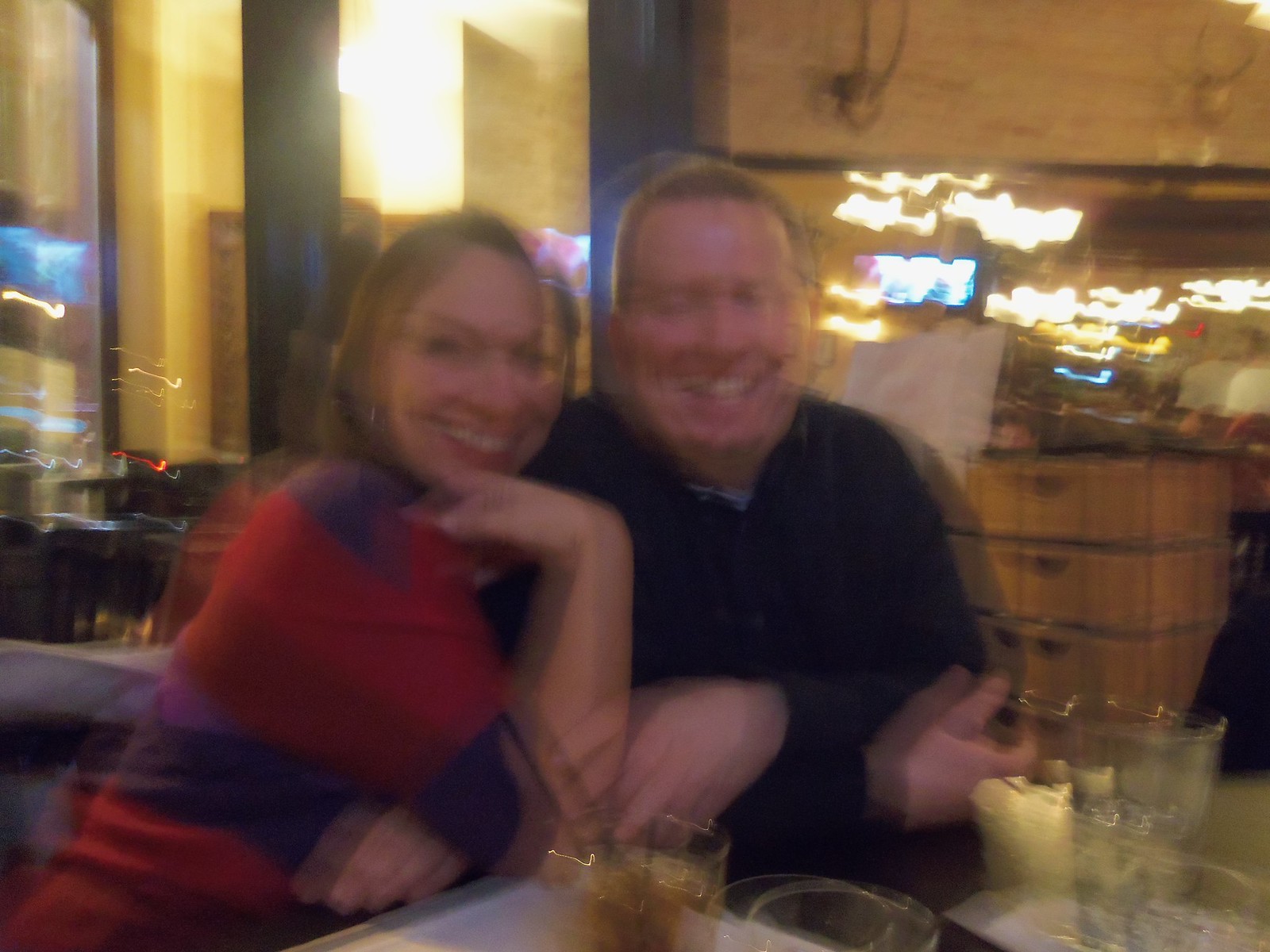In the blurred, out-of-focus photo, a couple is seated at a table adorned with drinks, presumably in a bar or restaurant setting. The photo captures a warm, yellowish-hued interior, with distorted, wavy lights in the backdrop due to camera shake. On the left, the woman, with shoulder-length blonde hair, is dressed in a red and black or possibly red and purple striped shirt. She leans slightly towards her partner with her chin resting on her hand, a broad smile lighting up her face. On the right, the man, sporting a dark shirt or jacket and short blondish hair, smiles warmly, his arms folded across and touching the woman’s arm. The scene around them features extensive woodwork and possibly signage, further hinting at the cozy, inviting atmosphere of the bar-like restaurant they're enjoying.